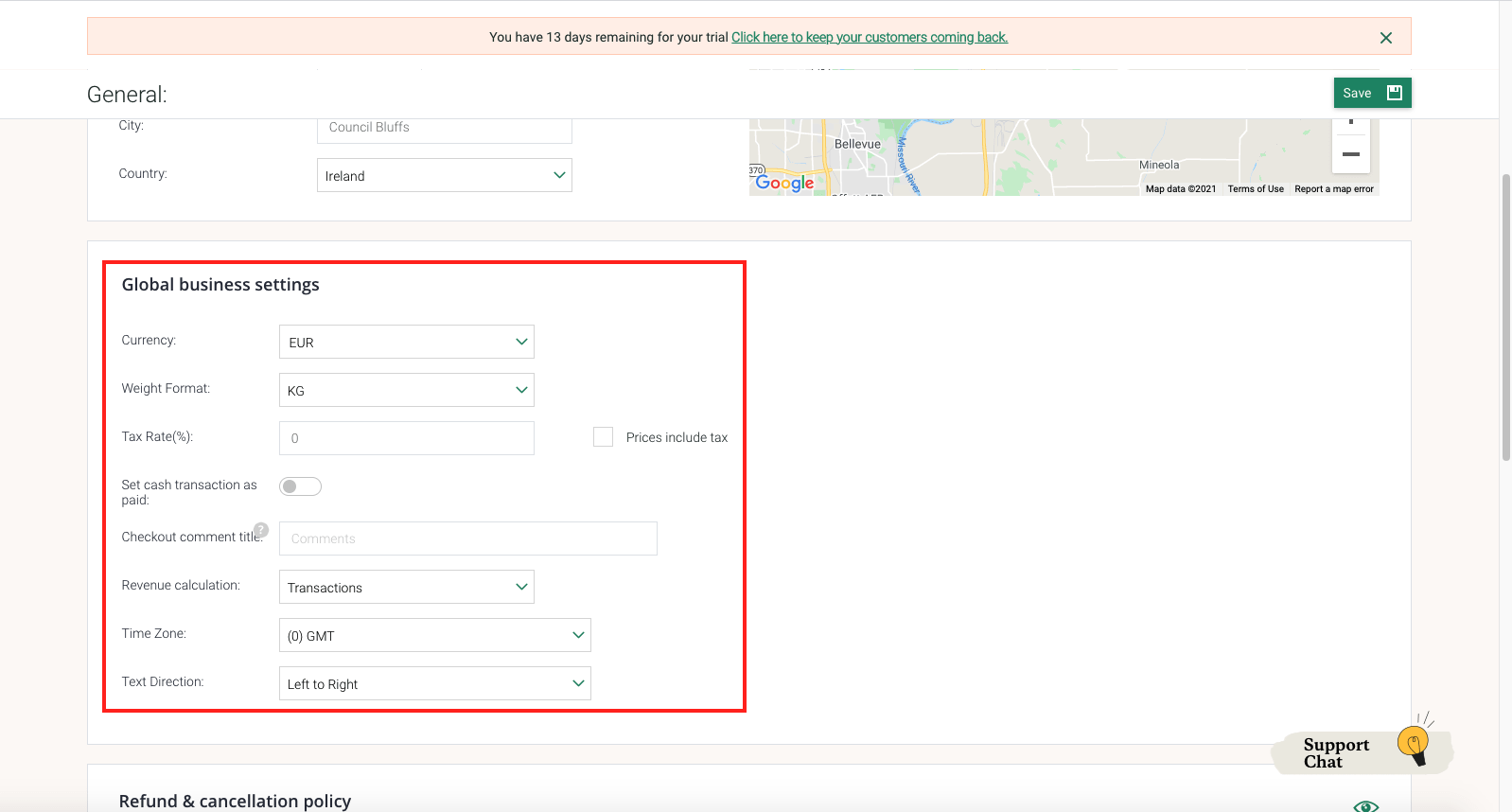Screenshot of a global business settings interface. A prominent red box highlights a section for focused attention, displaying a "Currency" drop-down menu currently set to "Euro." Adjacent to this, a "Weight Unit" marked as "kg" is visible. Although the "Tax Rate" field appears inactive, grayed out rather than blurred, there's a checkbox labeled "Price Includes Tax" which is not currently checked. Below, an option to "Set Cash Transaction as Paid" is displayed as a slider button positioned to the left. Further down, "Checkout Comment Title" is shown with a text field and a status of zero comments. 

Additionally, there's a "Revenue Calculation" section with a transaction type drop-down menu. The "Time Zone" setting, set to GMT, is adjustable through another drop-down box. The "Text Direction" option is set to "Left to Right," also changeable via a drop-down menu. 

At the top, a pink banner warns of 13 days remaining in the trial period, accompanied by a blue hyperlink encouraging continued customer engagement. The left sidebar contains general settings, where "City" is shown as Council Bluffs, grayed out, and "Country" is set to Ireland with modification options available. A partial map is visible at the bottom, about 20% of its display. In the bottom right corner, a "Support Chat" function, demarcated by a light bulb icon, is clearly labeled on two lines. To the bottom left, a bold text briefly reads "Refund and Cancellation Policy," hinting at further options beneath the visible interface.